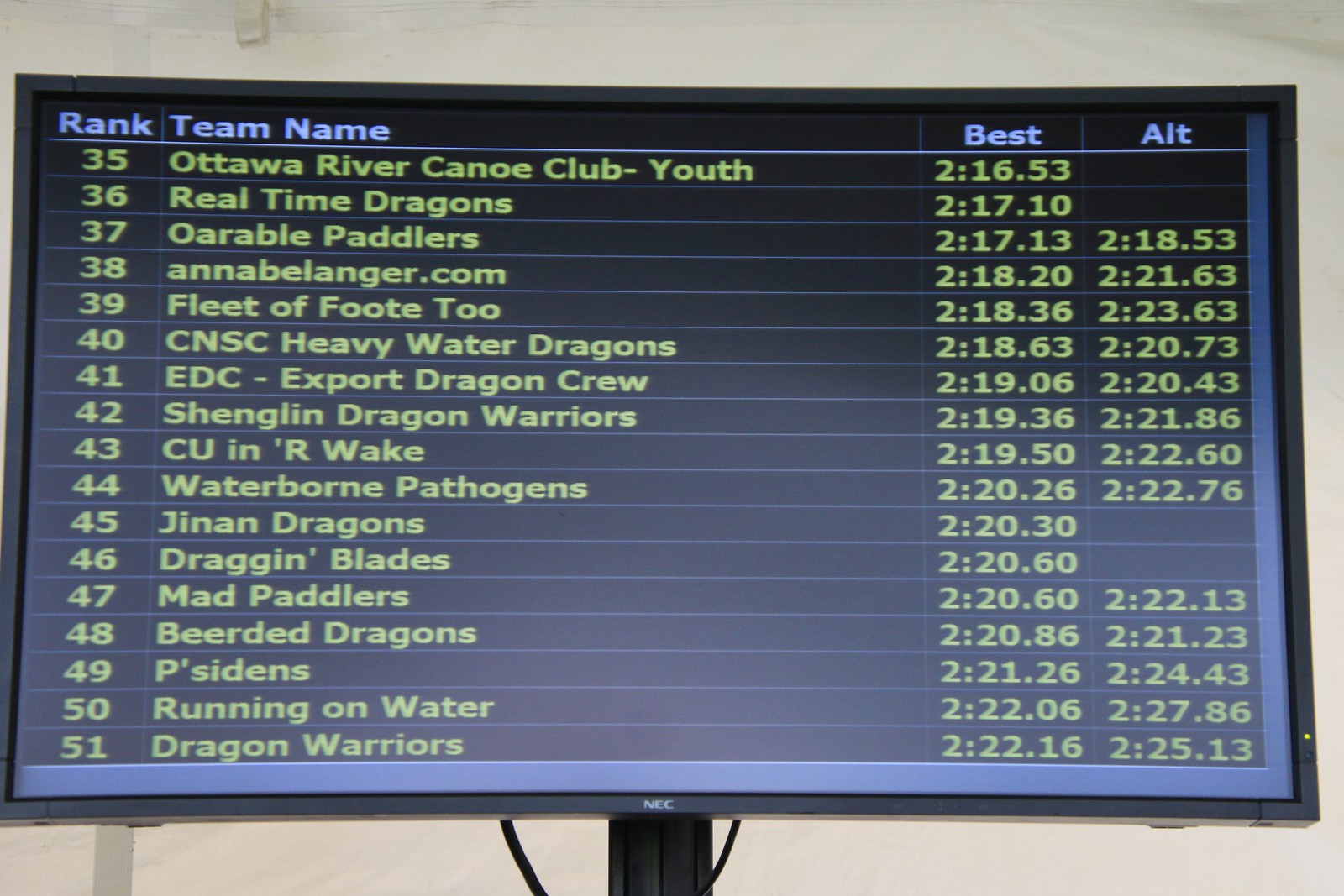The horizontal rectangular image showcases an electronic scoreboard, displaying rankings for a canoe race. The scoreboard, which appears on a black-framed NEC computer monitor mounted on a black stand, lists teams ranked from 35 to 51. The headings at the top are in blue, with three columns labeled: 'Rank,' 'Team Name,' 'Best Time,' and 'Alt Time.' The 'Best Time' and 'Alt Time' columns display the teams' recorded times. For instance, the Ottawa River Canoe Youth Club, positioned at rank 35, achieved the best time of 2:16.53, with no alternate time recorded. At the bottom, the Dragon Warriors, ranked 51, have a best time of 2:22.16 and an alternate time of 2:25.13. The screen is positioned against a plain white wall with no additional background detail visible.